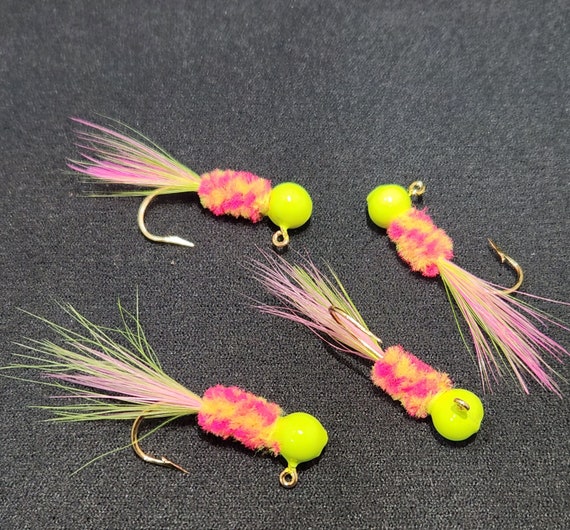This photograph showcases a set of four fly fishing lures, distinctly arranged against a dark gray fabric backdrop. Each lure shares a consistent design featuring a bright, neon yellow-green ball at the top, with a noticeable point for attaching the fishing line. From this ball extends a vivid mix of pink and yellow fuzzy material, giving way to artificial hair-like extensions in matching neon colors. These vibrant extensions are topped off with shiny, metallic silver hooks, equipped with barbs for capturing fish. The lures are haphazardly clustered in the center of the image, rather than being neatly aligned. Notably, two of the lures are facing upwards on the left side, while on the right side, one lure's hook points outward and the other upward, adding to the dynamic arrangement. The combination of neon pink and yellow colors against the dark background creates a striking visual contrast, highlighting the intricate details of the fishing lures.